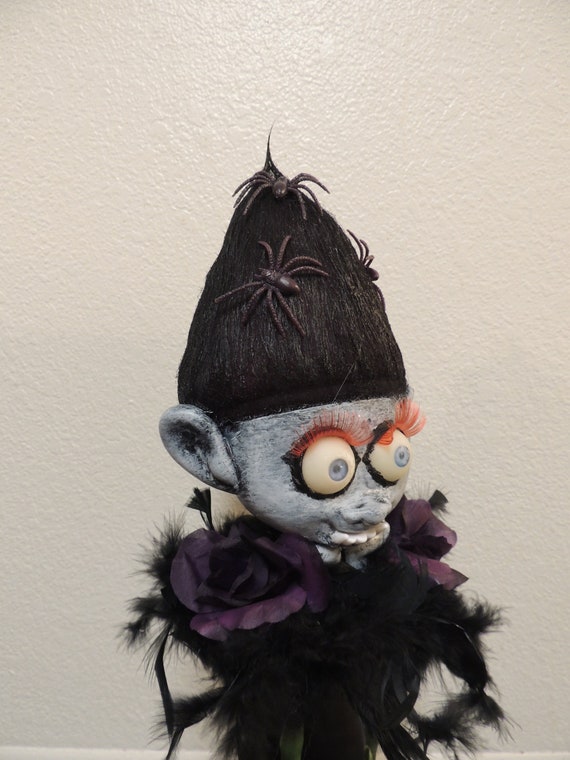The image depicts a handmade, alien-like creature with distinct, spooky features. The creature's face is gray, with large, bulging googly eyes that have prominent orange eyelashes. Its head sports very tall, black hair styled into a cone, atop which crawl three spiders. The creature's nose resembles a pig's snout, and its mouth displays several protruding lower teeth. Flanking its head are large, ear-like appendages. The body is covered in black feathers, adorned with an orange pattern and deep black-purple flower-like details on the shoulders. The background reveals a lightly textured wall in a cream or white color, providing a contrasting backdrop to the eerie figure.